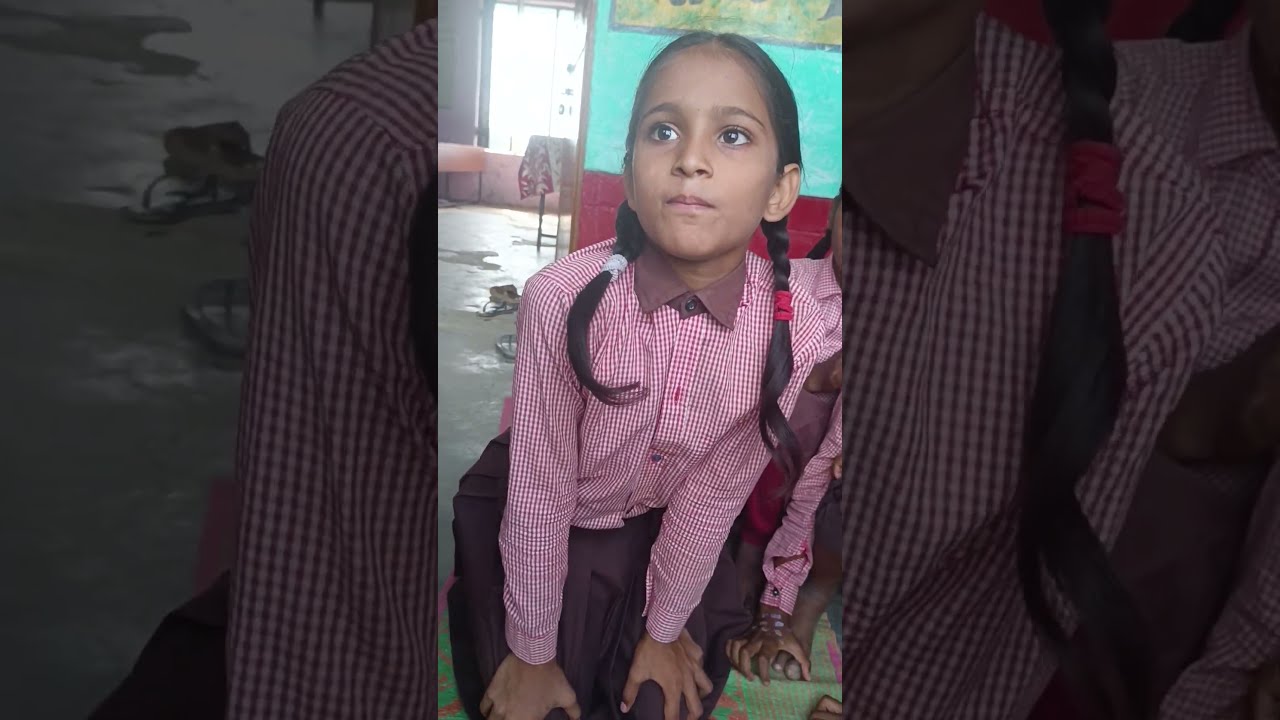A young girl with dark brown skin and black hair styled in pigtails that fall over her chest is looking up and to the left with a questioning expression on her face. She appears to be around six to eight years old and is wearing a red and white checkered button-down shirt, part of a school uniform, paired with dark pants. Her hands rest on her knees as she hunches forward slightly. Behind her, the background features a light teal wall with a darker red section at the bottom, and there is glare coming through a window. To the left and right are closeups, one of her left shoulder revealing a floor in the background, and another of her ponytail. The setting includes tables and a rug, suggesting an indoor environment, possibly a classroom. She gazes at something beyond the photographer, appearing curious, as if waiting for an answer to a question she might have asked.